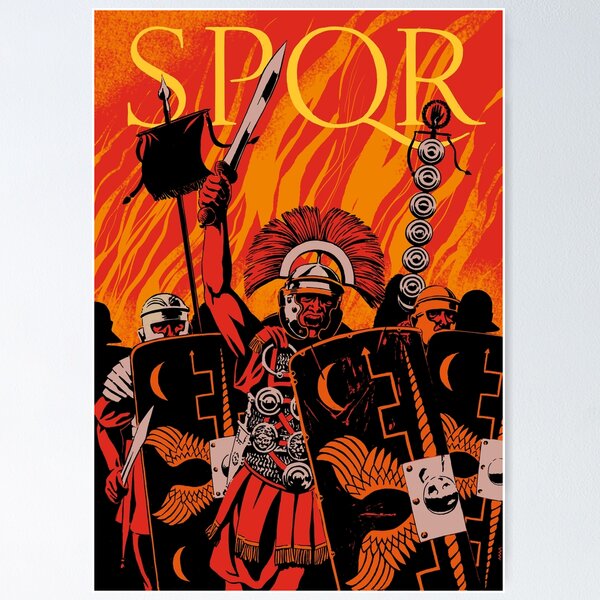The image is a vividly colored, graphic design-style poster with the dimensions resembling a book cover. At the top, in large yellow letters, it says "SPQR," which stands for the Senate and the People of Rome. The background is a fiery blend of reds, oranges, and yellows, giving the whole illustration a warm, war-oriented feel.

In the center of the image stands a commanding Roman soldier. He holds a silver sword aloft and appears to be yelling. His armor consists of chainmail and a skirt, and he wears a distinctive helmet adorned with red fur. His shield is black with yellow tribal and geometric designs including a moon, arrows, and wings.

To his left and right are two other soldiers, each partially obscured by their shields. The soldier to the left wears silver armor and helmet and has a silver sword pointed forward. The soldier to the right appears to have bronze armor and an orange helmet. Both have red skin, in line with the stylistic choices of the illustration. 

In the background, black silhouettes of additional warriors can be seen, adding depth to the scene. There is a flag featuring multiple black circles arranged along a pole topped with a hand symbol. This backdrop complements the intense, battle-ready atmosphere conveyed by the central figures.